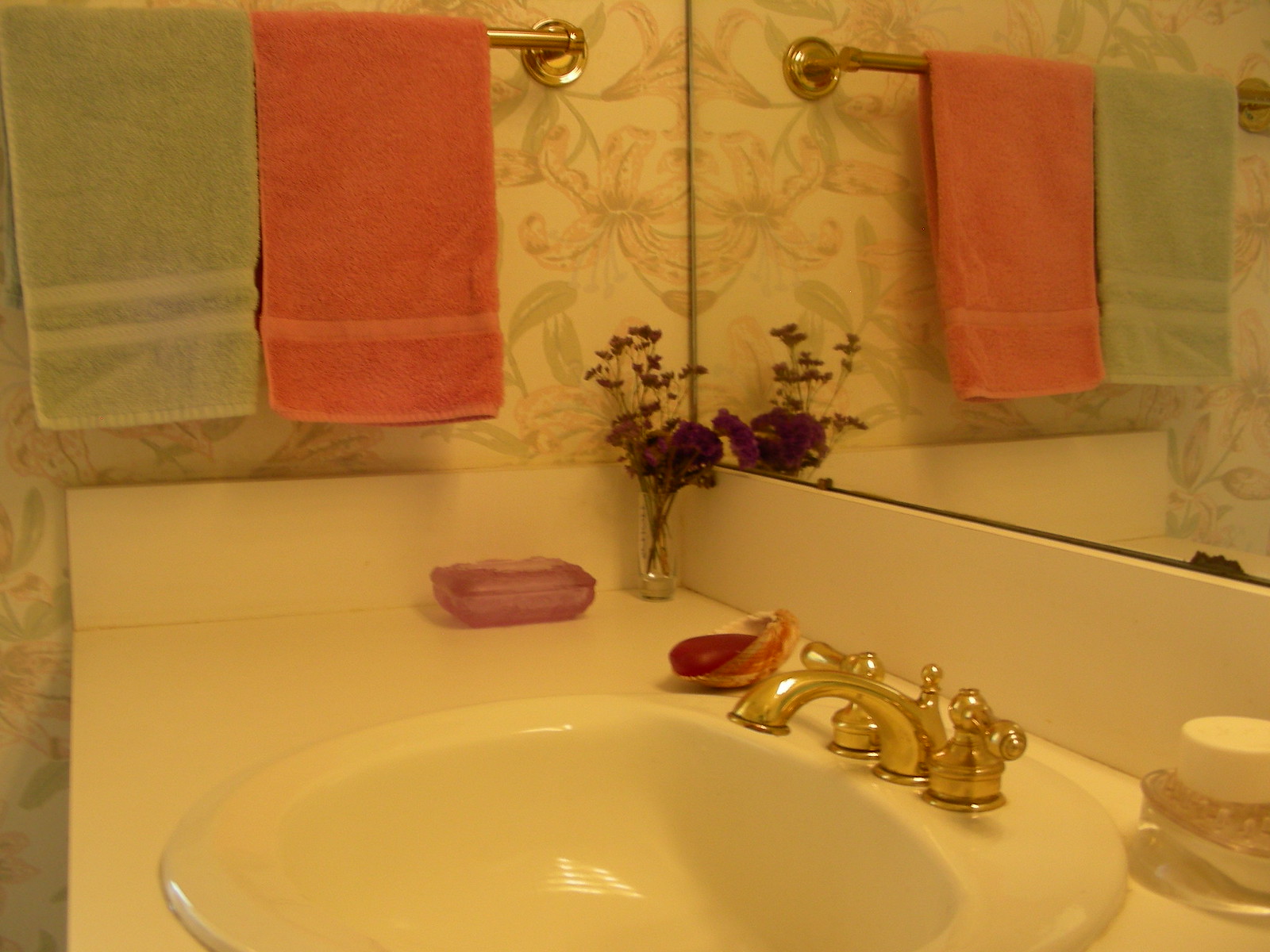A warmly lit bathroom countertop features a striking combination of functional and decorative elements. The sink, an oval white basin, is flanked by gold-tinted hot and cold water handles and a central spigot, exuding a touch of elegance. Anchoring the countertop is a tall, clear vase with delicate purple flowers, likely artificial, adding a pop of color and charm. Next to the vase sits a rectangular pink glass-covered bin, enhancing the countertop's aesthetic appeal. A large scallop shell sits adjacent, holding a bar of red soap, blending practicality with style. 

The wall facing us is adorned with a floral print wallpaper, providing a whimsical backdrop. A silver towel rack hangs on this wall, draped with a towel that appears greenish due to a yellow color cast—a photographic artifact distorting the presumed blue hues. The picturesque setting continues with a massive pane of mirror glass on the adjacent wall, reflecting the towel rack and expanding the space visually. To the far right, a clear air freshener with a perforated lid sits discreetly, adding a subtle touch of freshness to the room. The overall scene, despite the unnatural golden hue from the photo, captures a charming and well-appointed bathroom corner.